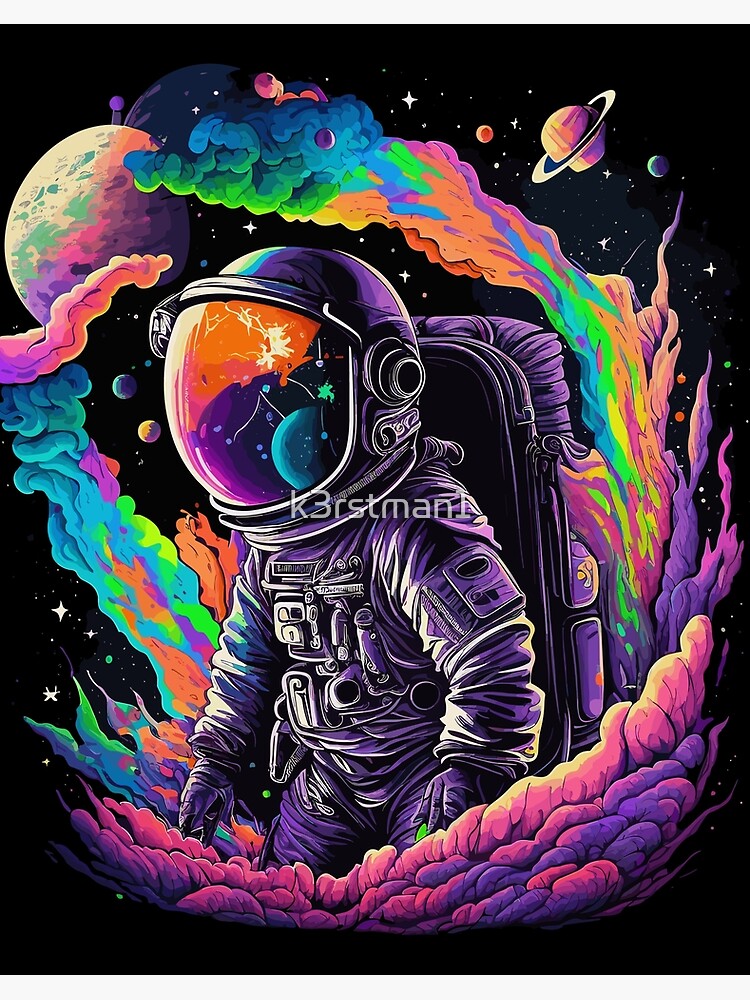In this vibrant, psychedelic artwork, a central figure of an astronaut is depicted amidst a cosmic, colorful spectacle. The astronaut, donning a light purple, wrinkled space suit complete with a huge, reflective helmet and a rectangular oxygen pack on their back, stands facing the left. The helmet visor reflects a surreal scene of a bright orange sky, a purplish landscape, and a blue-hued planet. The artwork is dominated by a chaotic yet mesmerizing array of colors: a cloud-like formation of pink, purple, lime green, blue, and yellow hues surrounds the astronaut, adding to the outer space theme with diverse planets and stars scattered throughout the black background. Notable celestial bodies include a planet resembling Saturn with its rings, and various colorful orbs in greens, oranges, and blues. The overall rectangular image is filled with white stars, depicted as tiny crosses, enhancing the deep space atmosphere. At the very center, horizontally across the artwork, is the text "K-3-R-S-T-M-A-N-1," possibly the artist’s signature. This vivid, surreal scene combines earthly astronautical details with fantastical cosmic elements, manifesting a truly unique piece of digital art.